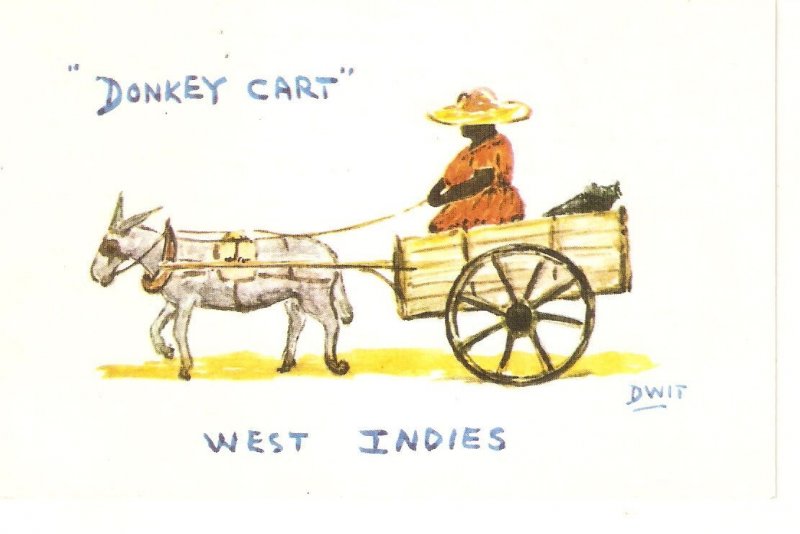This color illustration, possibly created with markers, features a quaint and simple scene from the West Indies. In the top left corner, the phrase "Donkey Cart" is written in light blue block letters and in quotation marks. Below the scene, also in blue, are the words "West Indies." The right side of the image bears the signature "DWIT," underlined in blue. The artwork depicts a one-wheeled cart being pulled to the left by a small, gray donkey with pronounced ears. The donkey, which appears to be wearing a bridle and yoke around its neck, has a serene expression and may be adorned with a mask or blinders. Seated in the cart is a large, dark-skinned woman dressed in a bright orange or red dress. She wears an expansive yellow sun hat, and behind her in the cart, there's a dark-colored bag. Holding the reins, she guides the donkey along a surface that suggests a yellow road. The entire scene exudes a charming, simplistic beauty reflective of its exotic locale.